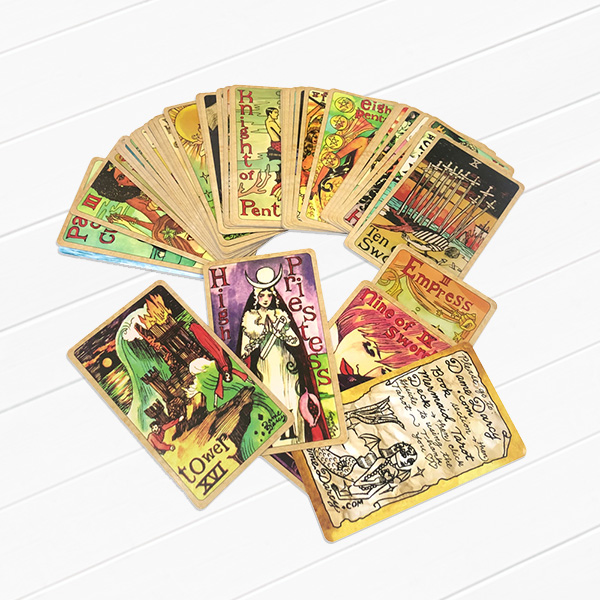The image features a photograph of a tarot deck spread out on a white surface with diagonal blue lines running from the bottom left to the upper right. The cards are partially fanned out in a semicircular pattern, revealing an intriguing array of detailed illustrations and text. Among the prominent cards, there's one depicting a man on his hands and knees crawling toward a castle with the title "Tower XVI" in Roman numerals, suggesting the Tower archetype. Another card displays a woman in a white gown with a quarter moon and a circle above her head, labeled "High Priestess." Additionally, the Empress card is visible. The cards exhibit various vibrant colors and appear slightly worn out, perhaps intentionally aged, with brownish tints, but their edges remain intact. The overall display offers a captivating glimpse into a well-illustrated tarot deck.